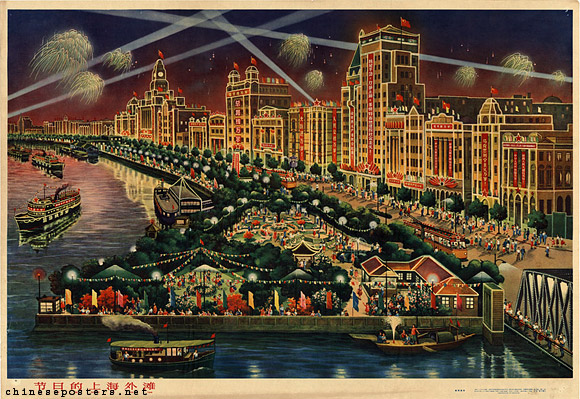This image, sourced from ChinesePosters.net, is a vibrant and detailed drawing reminiscent of an old postcard or promotional poster. It captures a bustling, celebratory cityscape by the sea during nighttime. The colorful scene portrays a lively atmosphere along a broad walkway lined with various restaurants and shops, their bright advertisements visible on the buildings above. These buildings, which seem to have shops on the lower levels and apartments on the upper, are bathed in light, creating a festive mood. 

People are depicted enjoying themselves, strolling along the street and the broadwalk, which is bustling with activity. The broadwalk overlooks a serene body of water—possibly a canal, river, or lake—filled with large ferry boats and barges that host houses or shops. Along the walkway, trees and brightly colored lights strung from metal poles add to the festive ambiance. 

In the backdrop, the sky is alive with fireworks and crisscrossing spotlights, enhancing the celebratory feel of the scene. This richly detailed artwork captures the essence of a joyful time in a vibrant city by the sea.